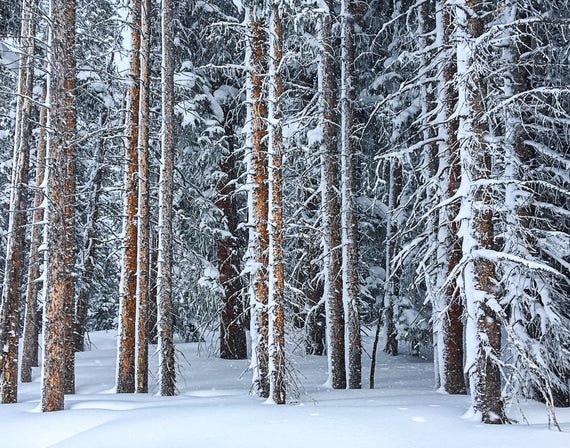This image appears to be a digital render or painting of a winter forest. The scene is dominated by very tall, thin trees with golden brown to dark brown trunks, some of which have a subtle gray hue. The branches are completely bare, covered in a pristine layer of snow. The ground is also entirely blanketed in undisturbed snow, except for a few spots and footprints visible among the trees, suggesting minimal activity. The trees are densely packed, leaving little room for the sky to be visible, other than at the very tops in sparse gaps. The serenity and cleanliness of the snow-covered landscape further indicate that this is likely a digital creation rather than a real photograph.